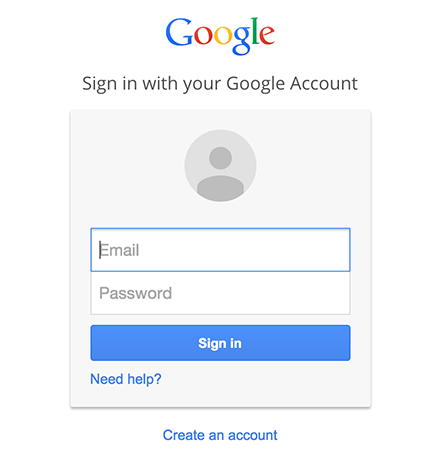A screenshot of a Google sign-in page displayed on a device, possibly a laptop, is shown. At the top of the screen, there is the iconic Google logo, featuring its multicolored letters. Directly below the logo, there is a prompt to "Sign in with your Google account." The main section of the page features a light gray dialog box prompting the user to enter their credentials. At the top of this box is a circular placeholder image in dark gray, representing a user's profile picture. Below this, there are input fields: one for entering an email address, currently blank with the cursor placed inside, and another for entering a password. Both input fields appear in medium gray. Below the password field, there's a blue button with white text labeled "Sign in." For users who need assistance, there is a "Need help?" hyperlink in blue text right below the sign-in button. Lastly, for those who do not yet have a Google account, there is an option to "Create an account," also in blue text, situated at the bottom of the dialog box. The overall layout and design are clean and functional, characteristic of Google's user-friendly interface.